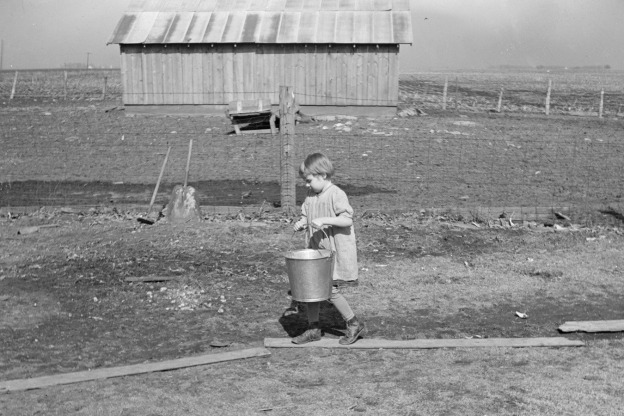This black and white, horizontally aligned photo captures a young girl with short blonde hair walking to the left across narrow wooden planks laid over muddy ground on a farm. She wears a baggy, light-colored dress with black shoes or boots and leggings. She carries a metal bucket by its handle, and her path is bordered by grass and dirt. A barbed wire fence supported by wooden posts runs across the middle of the image, behind which there is a farmyard with dirt, rock, and a rectangular building with a hipped, possibly metal, roof, and made of wooden panels. Leaning against this fence are a shovel and a push broom. The scene is set under a sky filled with gray clouds.